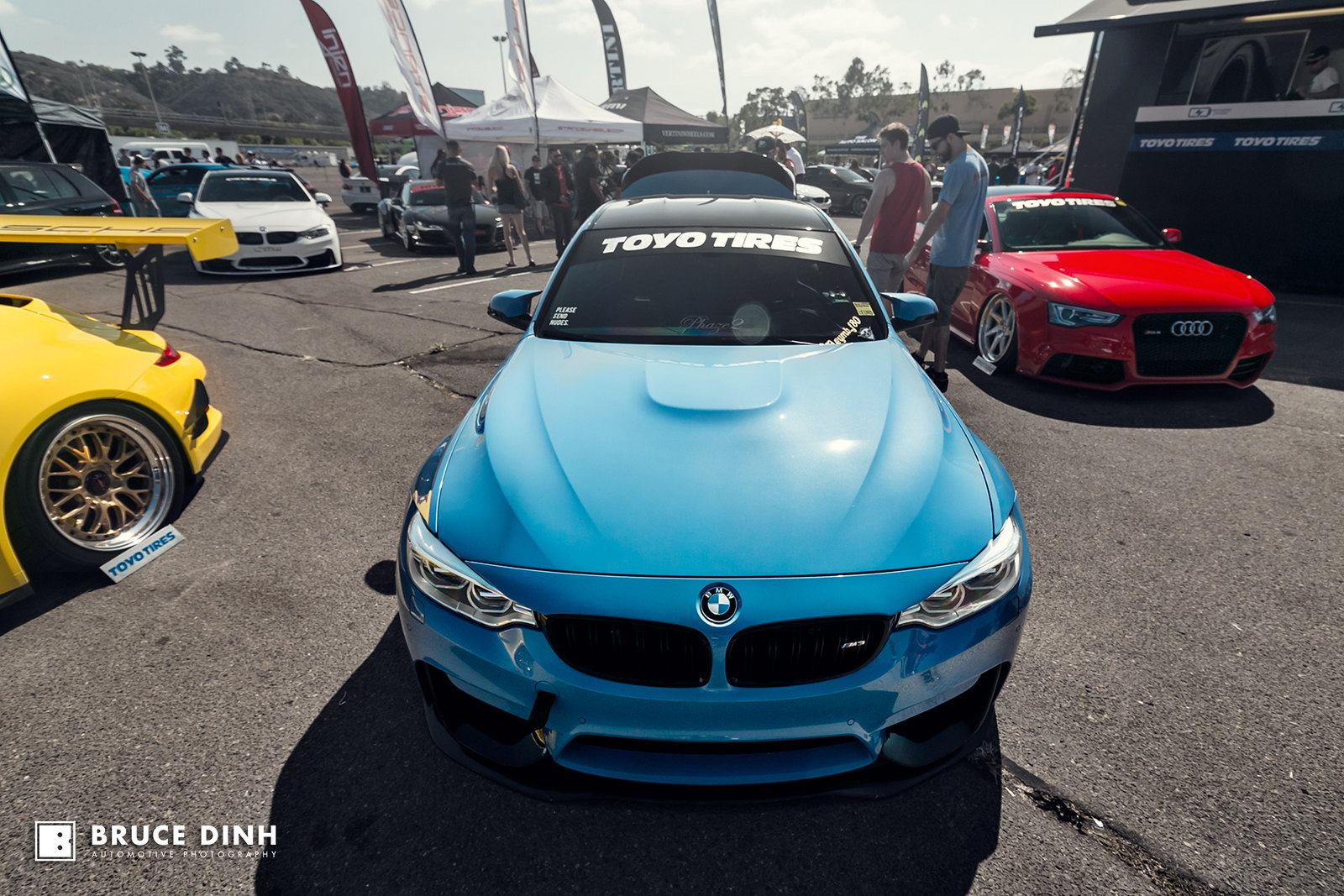This is a color photograph taken outside on a sunny day, capturing a vibrant parking lot filled with high-end, modified cars likely showcased for a Toyo Tires event. The central focus of the image is a bright medium blue BMW facing directly at the camera, with "Toyo Tires" displayed prominently across the top of the windshield in large white block letters. To its left, the rear section of a bright yellow car with a spoiler can be seen, sitting low to the ground. To the right and slightly further back is a bright red Audi, also featuring the "Toyo Tires" branding on its windshield. The scene is bustling with activity; two young adult males in summer attire are walking among the cars, while larger groups of people and more vehicles are visible in the background. Additional cars from various brands—including BMWs, Mercedes, and Toyotas—all bear the Toyo Tires branding, with corresponding signs near their tires. Flags and a building adorned with the Toyo Tires logo further emphasize the theme of the event. At the bottom left corner of the image, the watermark reads "Bruce Den Photography."